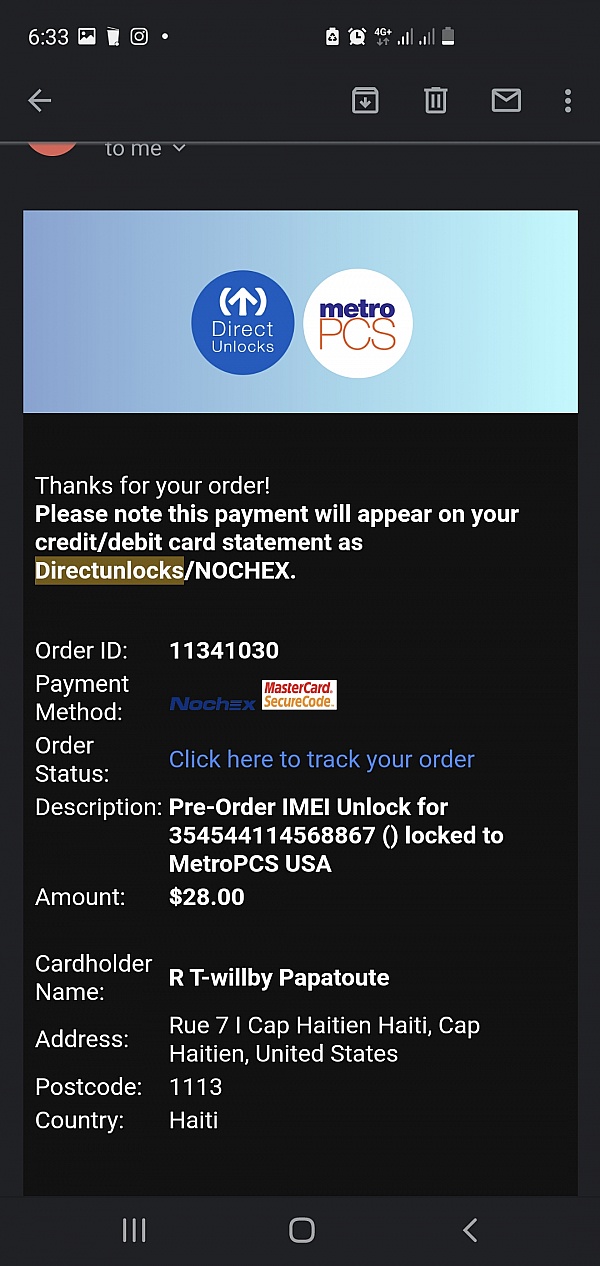Captured from a cell phone screen at 5:33 with a nearly full battery, the image showcases a payment confirmation page. At the top, a small gray arrow points left, followed by a long line, and then a blue square. The square transitions from a slightly grayish blue on the left to a light blue on the right, with a central blue circle labeled "DIRECT" and an upward-pointing arrow.

To the right of this icon, there is a white square displaying "METRO PCS" in uppercase letters. Below, a message thanks the user for their order and informs them that the payment will appear on their credit/debit card statement as "DIRECT LOCKS," highlighted in dark yellow, followed by "- CHEX."

Further details include:
- Order ID: 1134130
- Payment Method
- Order Status
- Description
- Amount: $28

Additional information listed includes:
- Cardholder Name
- Address
- Postcode
- Country: Haiti (H-A-I-T-I)